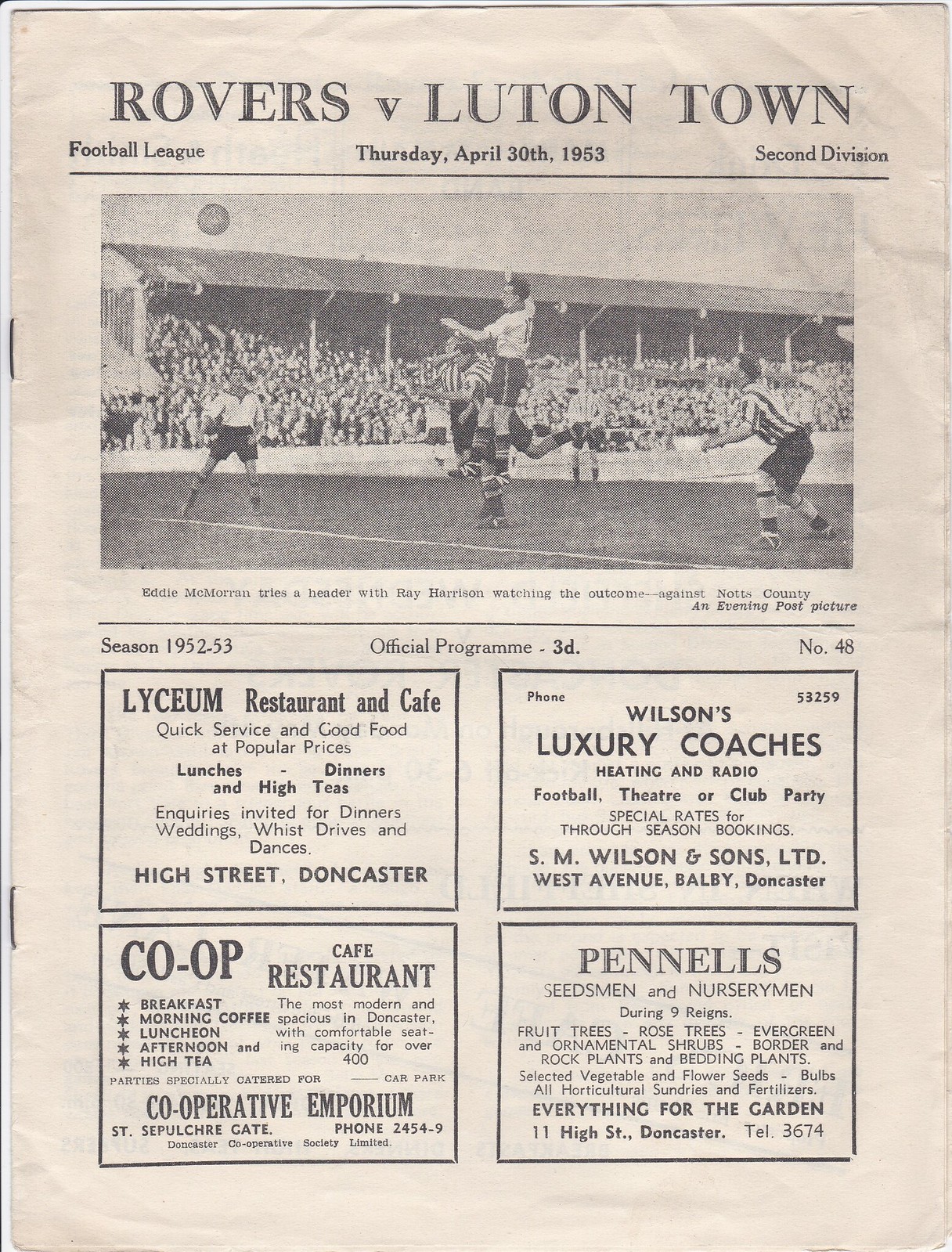This image depicts the front page of an old British football (soccer) magazine from 1953, which serves as a program for a match between Rovers and Luton Town. The background is white, and the magazine is bound with staples on the left-hand side. At the very top, in a bold black font, it reads "Rovers v. Luton Town," with additional details underneath in smaller black text: "Football League" on the far left, "Thursday, April 30th, 1953" in the center, and "Second Division" on the right. 

A thin line separates this section from a black-and-white photograph capturing a dynamic moment in the soccer match, where a player, identified as Middle McMorrin, attempts a header while Ray Harrison watches the outcome. The photograph is credited to an "Evening Post picture." Below the photograph, another thin line runs across the page, followed by the text "Season 1952-53" on the left, "Official Program 3D" in the center, and "Number 48" on the right.

Below this text are four neatly boxed advertisements: the Lyceum Restaurant and Cafe, Wilson's Luxury Coaches (which also mentions heating and radio services), Co-op Cafe Restaurant, and Panels, Seedsmen, and Nurserymen. The vintage design and the content of the program give it a nostalgic feel, reflecting the era's typical match-day memorabilia.